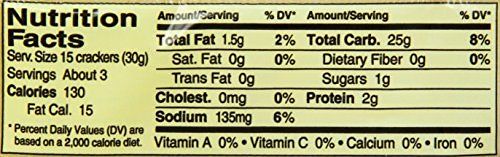This image showcases the nutritional facts label of a food product, likely crackers, as indicated by the serving size listed. The label itself is displayed on a rectangular, yellow background with a black outline, featuring black text for contrast. The nutritional information includes detailed values for total fat, saturated fat, trans fat, cholesterol, sodium, and carbohydrates, among other elements. Specifically, the label notes that one serving size consists of 15 crackers, with about three servings per container. Each serving provides 130 calories, 15 of which are from fat. Additionally, the label lists vitamins and minerals, showing 0% for Vitamin A, Vitamin C, Calcium, and Iron. Percent daily values are provided for each nutritional component, along with descriptions to clarify the abbreviations and their significance in the context of a daily diet. This comprehensive label offers consumers a thorough understanding of the nutritional content and health implications of the product.